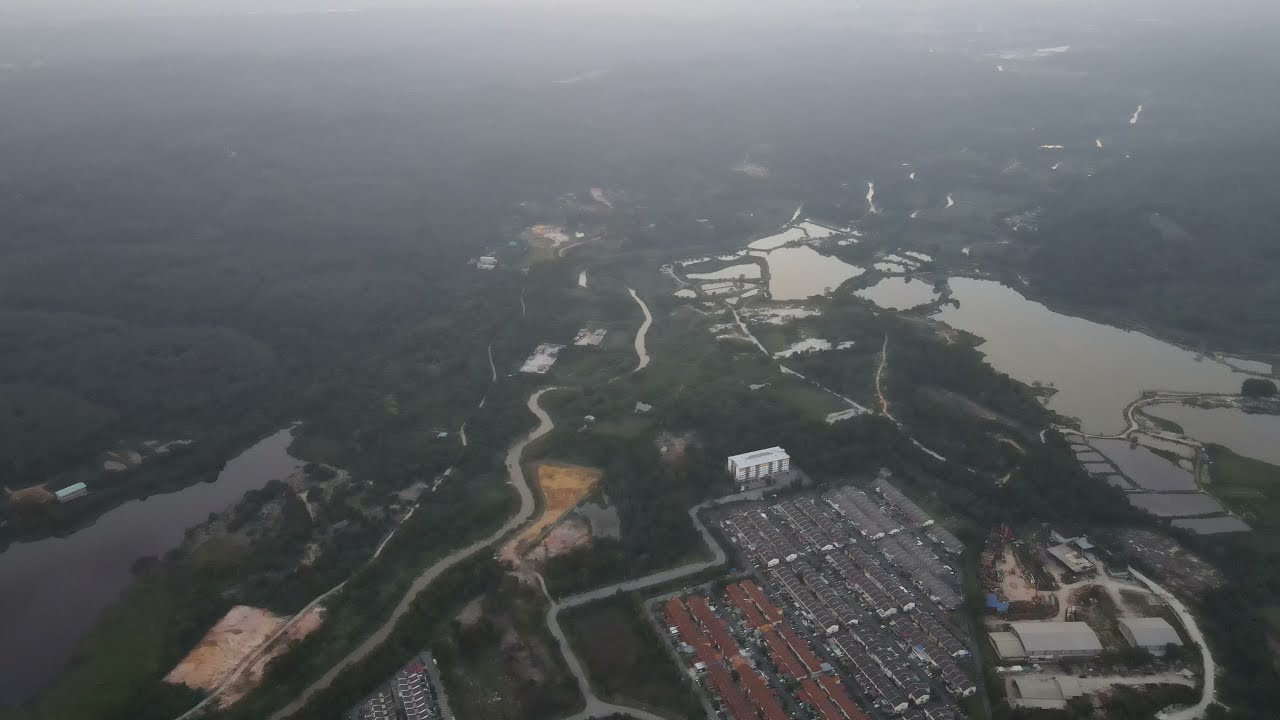This photograph, taken from the sky, features a hazy aerial view of a misty and foggy landscape. Central to the image are two lakes, connected by a winding river nestled within a shallow valley between gently sloping, green hillsides. Between these lakes and river lies a large, paved area densely populated with rows of houses, displaying a mix of red and gray roofs. A white apartment building stands out at the end of one of these rows. The right side of the image is dominated by an industrial complex, including a group of larger factory-like buildings. The surrounding area is lush with trees, resembling a forest, and spiral-shaped roads weave through the landscape. Natural bridges formed by trees and green areas divide the larger bodies of water, adding to the intricate tapestry of the scene. The image is devoid of people, emphasizing the tranquil, uninhabited atmosphere.